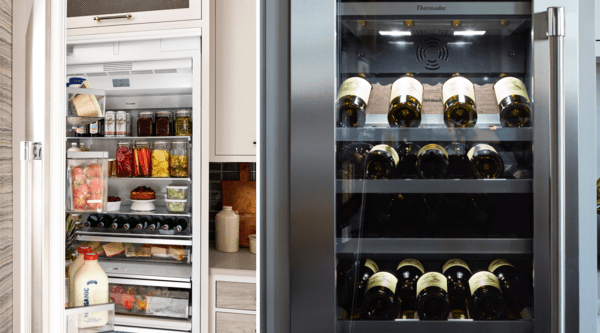This is a detailed photograph of a modern kitchen, carefully staged to showcase its organization and aesthetic appeal. The image is a collage featuring two distinct refrigerators. On the left side, there's a pristine white kitchen refrigerator with its door open, revealing well-organized shelves. The door compartments contain bottles of milk, while the interior shelves are meticulously arranged with containers of vegetables, fruits, kimchi, and pickles. Several shelves are dedicated to neatly laid out beer cans, adding a colorful and symmetrical touch. On the right side, there is a sleek, silver wine cabinet with a transparent glass door. This wine cooler boasts 14 bottles of wine, evenly distributed across the shelves, and illuminated by an integrated lighting system. The cabinet's polished, reflective surface complements the rest of the kitchen's sophisticated design. Adjacent to the wine cooler on the right are additional kitchen cabinets and drawers, with a counter adorned with a small vase and other decorative items. The backsplash features brown tiles, enhancing the warm and inviting atmosphere of the kitchen.